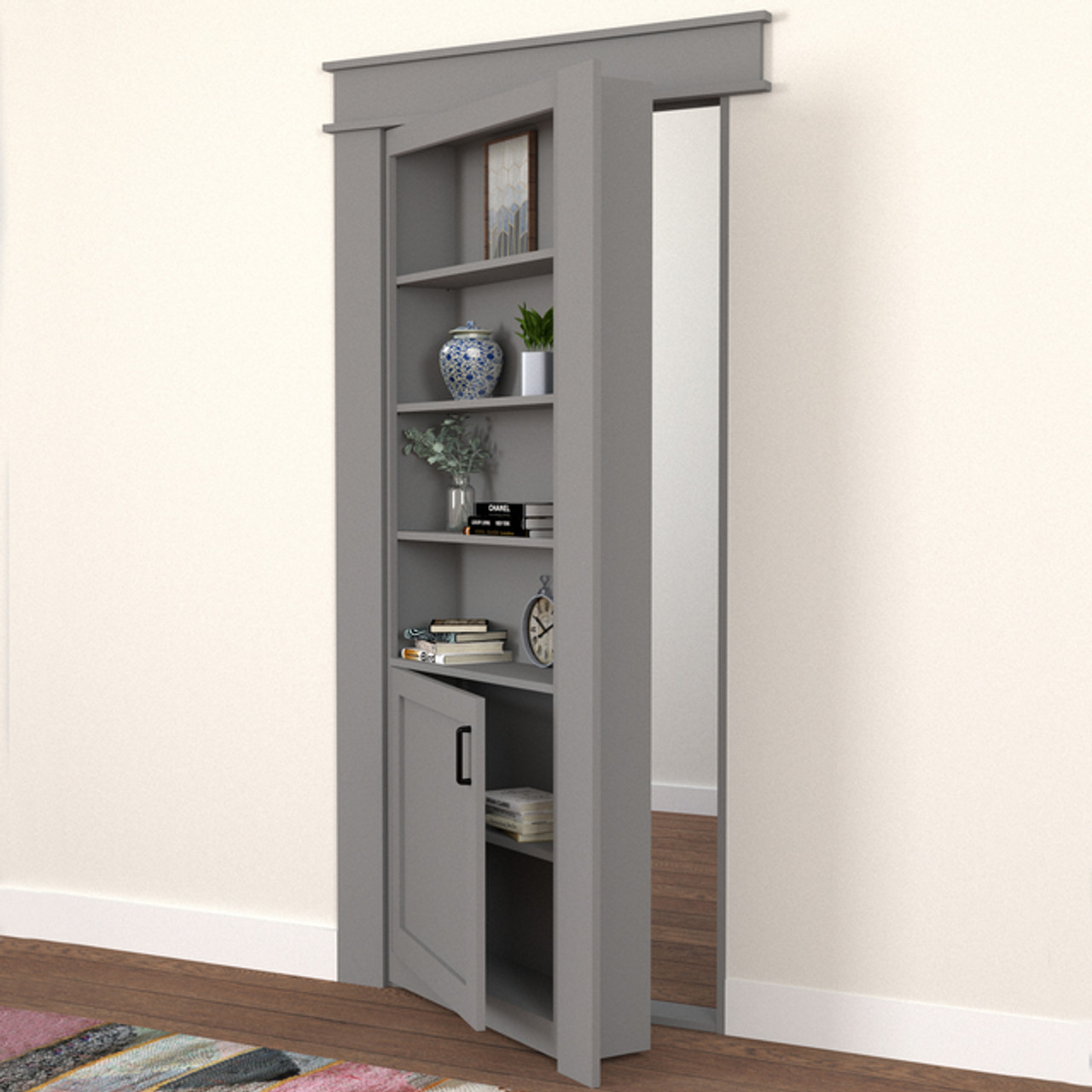The image depicts a cleverly designed hidden door that doubles as a shelving unit, set in an indoor room with white walls and dark brown wooden flooring. The picture is taken at an oblique angle, roughly 45 degrees, highlighting the door's subtle integration into its surroundings. The door itself is slate blue and framed by similarly colored headboards and sideboards, making it nearly indistinguishable from a standard cabinet when closed. 

The shelving unit features four open shelves and a cupboard at the bottom. The top shelf holds a framed photograph or painting. The second shelf houses a vase and a plant. The third shelf contains another vase, some books, and possibly a jar. The fourth shelf has a stack of books and a clock. The cupboard at the bottom, which is slightly ajar, reveals additional books. Beside the door, the room has a multicolored rug with shades of white, black, pink, and blue located in the bottom left-hand corner of the image. Through the ajar door, another room is visible with similar wooden panel flooring and a white wall.

The intriguing aspect of this design is its dual functionality as both a door and a cabinet, blending utility with aesthetic appeal. The door appears to lack a conventional handle, possibly using a latch mechanism to open and close.